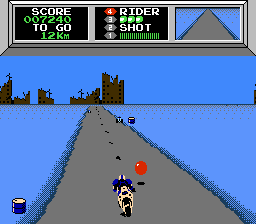In this screen capture from a racing video game, we see a first-person perspective of a man on a motorcycle speeding down a gray road that fades into the horizon. The road is flanked by a featureless blue void on either side and is marked with black dots down the center that suggest lanes. In the distance, the ruins of a blackened, post-apocalyptic city loom ominously. Hovering slightly above the road ahead of the rider is a red ball, seemingly an in-game objective or obstacle. The motorcycle rider is equipped with a helmet and is dressed in a blue shirt. Off to the left side of the road, there is a solitary barrel. At the top of the screen, score boxes display player stats: a score of 7,240 and a remaining distance of 12 kilometers. Additional statistics labeled "rider" and "shot" are also visible, indicating gameplay elements related to the rider's performance and actions.